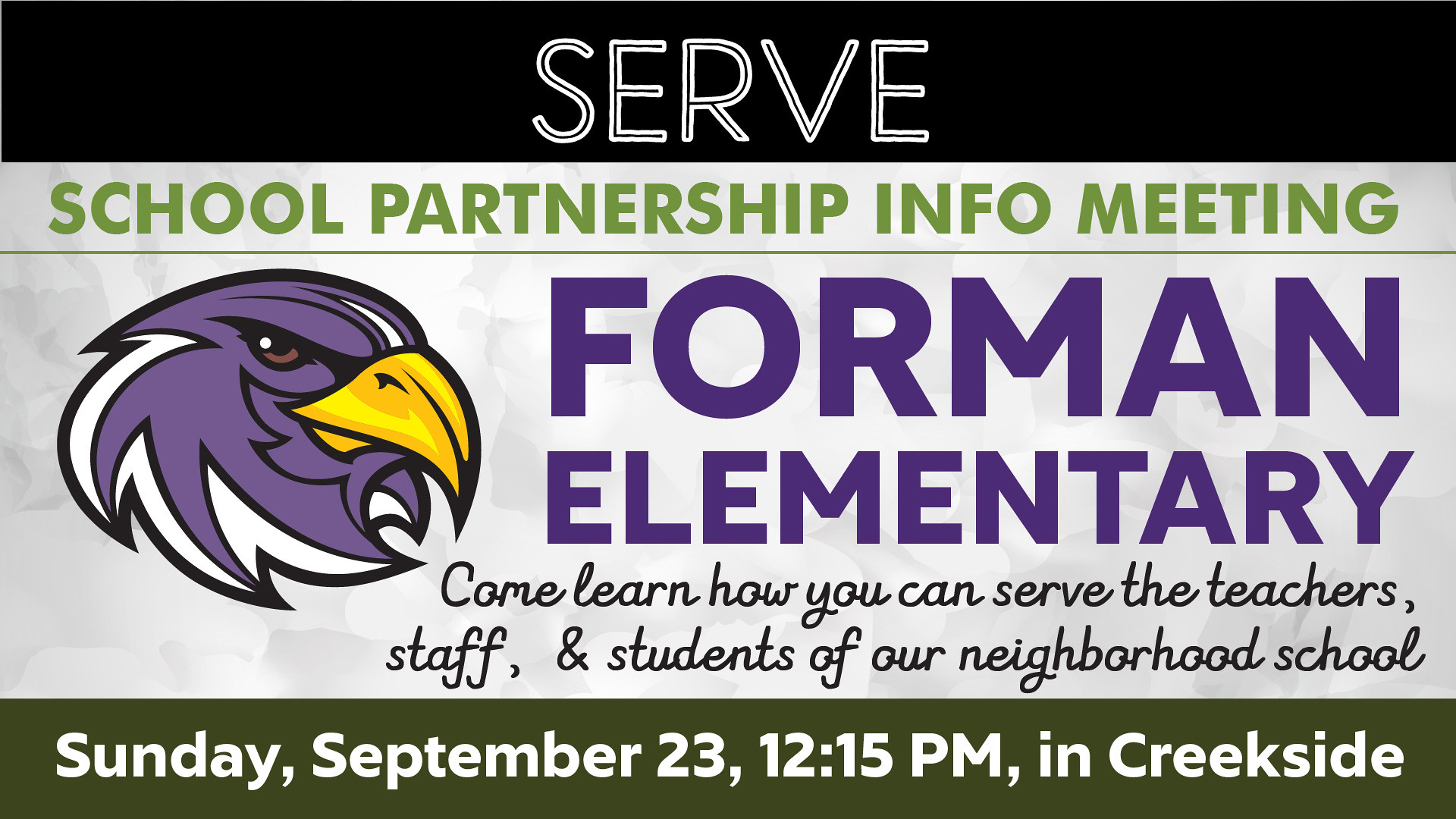This digital announcement, likely for Foreman Elementary, features prominent white text outlined in black at the top against a black background, reading "SERVE." Below that, in green letters, it states "School Partnership Info Meeting." On the left side, there is a stylized purple eagle head with a yellow beak, red eyes, and white feathers, probably the school mascot. To the right of the eagle, in large purple letters, it reads "Foreman Elementary." Below this, in black cursive writing, the text invites readers to "come learn how you can serve the teachers, staff, and students of our neighborhood school." The bottom section, set against a brown-green background with white lettering, provides the details: "Sunday, September 23rd, 12:15 p.m. in Creekside."